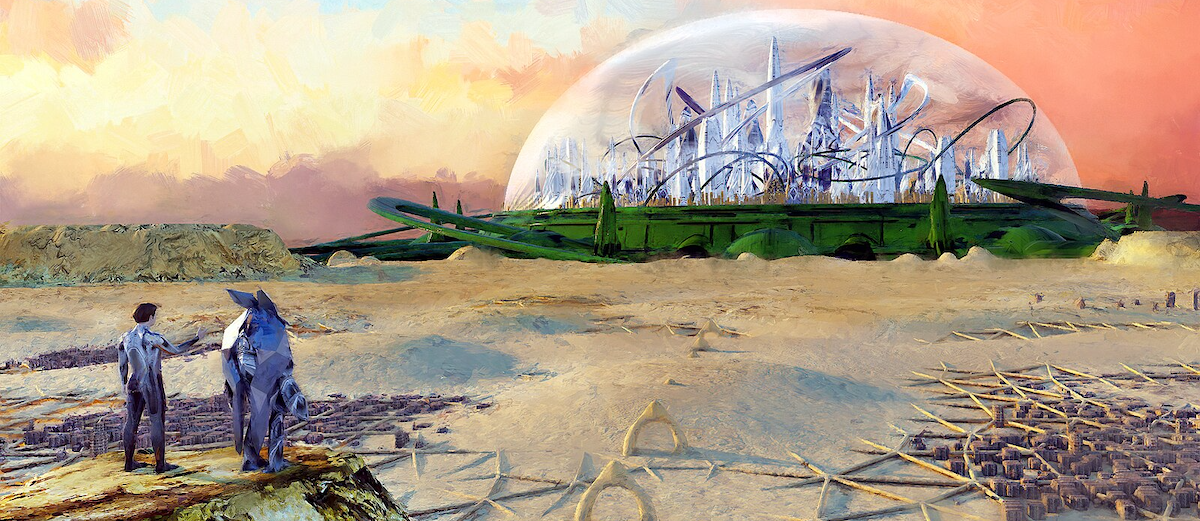The digital art image depicts a futuristic city encased in a glass dome in the upper right quadrant. The sky surrounding the dome transitions from pale orange to a blend of blue, yellow, and brown, producing a watercolor effect. The city within the dome appears advanced and bustling, reminiscent of a Jetsons-style metropolis, filled with swirling lines, intertwining tracks, roller coaster-like trails, and tall buildings. At the dome's base is a green structure resembling a boat or space shuttle, with intricate twisty designs and spaceships.

In the foreground, on the lower left, three figures stand on a sandy, tan and blue-ground landscape, with organized debris, including narrow crisscross yellow objects and purple rocks, scattered in the lower right corner. One of the figures is a man pointing towards the city, dressed in a simple shirt and pants. Another figure, standing nearby, wears a gray suit. Close to them, a third figure, an anthropomorphic creature dressed in blue armor with giant ears, gazes at the futuristic city. The scene evokes a blend of science fiction and fantastical elements, capturing a meeting of the old and new worlds under a surreal, dreamy sky.